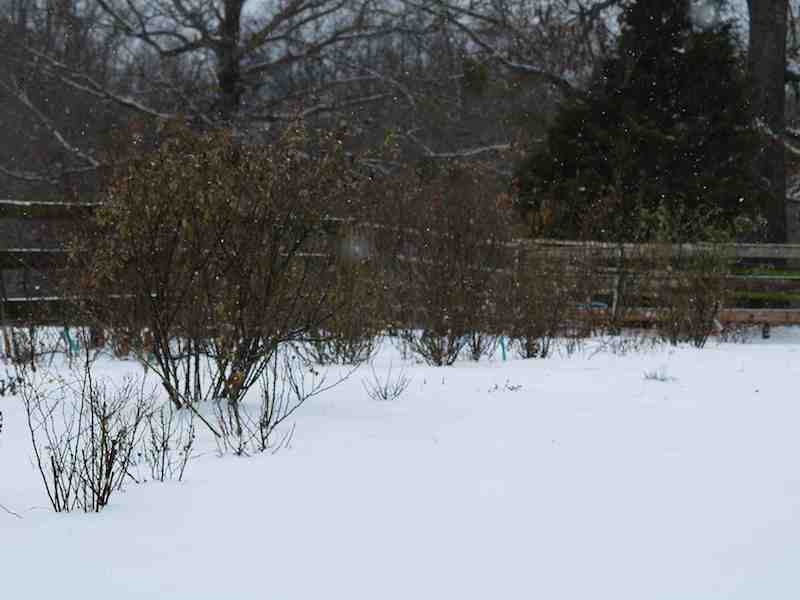This color photograph captures a serene wintery landscape. The foreground is blanketed in pristine white snow, creating a crisp, peaceful ambiance. Midground, there is a brown wooden fence composed of posts with three horizontal planks, partially obscured by dried brown bushes and brush, characteristic of winter's bare splendor. Several bare trees populate the background, their stark branches silhouetted against the dim sky. Notably, on the right side of the image stands a small, green evergreen tree that retains its foliage despite the season. Snowflakes gently descend, adding a dynamic element to the otherwise still scene. There's an absence of people, animals, vehicles, and text, allowing the viewer to fully immerse in this tranquil, undisturbed moment.